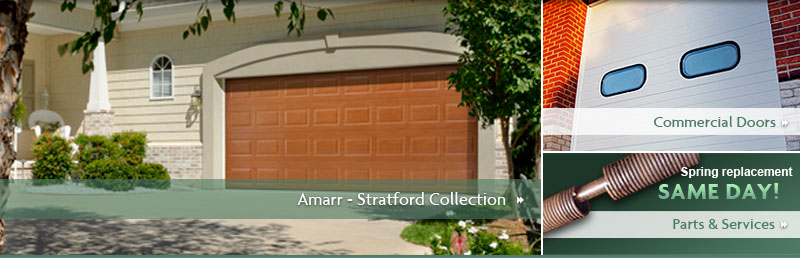**Amar Stratford Collection Advertisement: Premium Garage Door Solutions**

On the left side, the main image showcases the elegant exterior of a house with pristine white siding and a stylish garage door in a warm orange-brown hue. Superimposed over this image is a semi-transparent green background with the text "Amar Stratford Collection" in crisp white font, emphasizing the premium quality and design of the garage door.

In the top right, a smaller image features a business garage door with two small panels centered in the middle. The garage is set within a brick building, and the door itself is a clean, white color. This image has an overlay with a white transparent background, displaying the words "Commercial Doors" in bold green text, signifying the product's versatility for commercial use.

At the bottom, a detailed image of a garage door spring is presented, highlighting the service aspect of the advertisement. Accompanied by text that reads "Spring Replacement, Same Day," it emphasizes the company's prompt service. Below this, the text "Parts and Services" is highlighted, guiding customers to further information on available services.